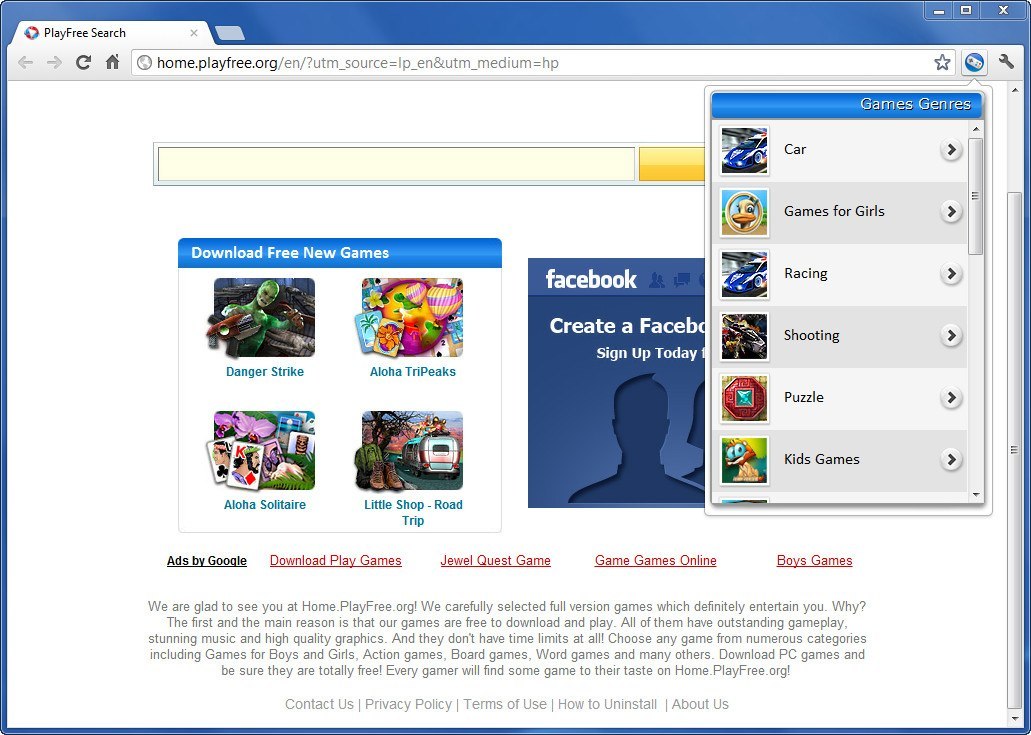The image is a screenshot of a web page titled "Play Free," reminiscent of the Windows XP or Vista era. The web address bar displays "home.playfree.org/EN/?UTM_source=LP_EN&UTM_medium=HP". Below the address bar, there is a search bar accompanied by a yellow search button, with a pop-up box located to its right.

At the top of the web page, a blue bar titled "Games Genres" is prominently displayed, followed by a list of various game genres such as car games, games for girls, racing, shooting, puzzle, and kids games. Each genre has a rightward arrow indicating further navigation options, and a scroll bar is available for additional selections.

To the left, another blue bar reads "Download Free New Games." This section showcases several game titles with accompanying images: "Danger Strike" featuring a zombie holding a gun, "Aloha Tri Peaks" with Hawaiian symbols, "Aloha Solitaire" under a Hawaiian theme, and "Little Shop Road Trip" with visuals of a car, boots, and a tree.

There is also a box that promotes Facebook, urging users to "Create a Facebook account, sign up today." This box is blue and contains outlines of people. Below this section, extensive text is visible with references to advertisements and downloadable games, such as "Ads by Google," "Download Play Games," "Jewel Quest Game," "Games Online," and "Boys Games." Additionally, there is a message about site usage included in this text-heavy area.